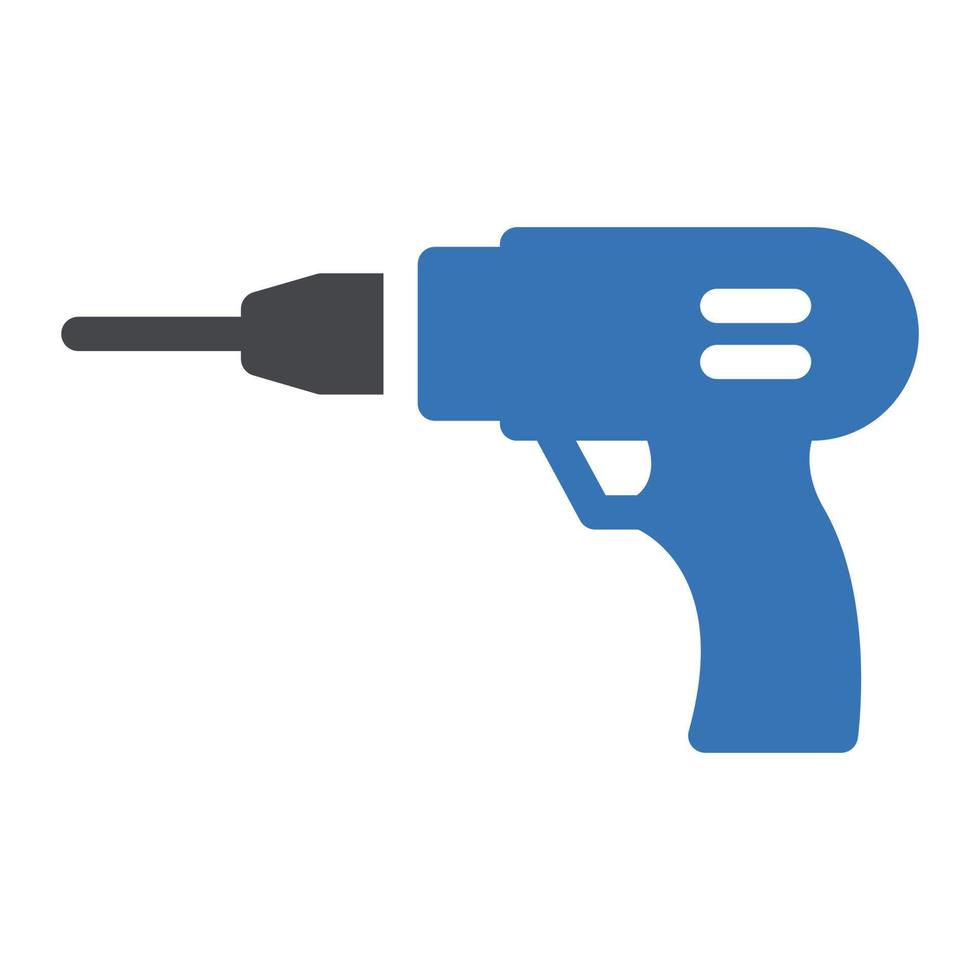The image is a stylized, 2D representation of a drill set against a stark white background. The body of the drill is depicted in a grayish-blue color, featuring a handle with a slight curve designed for ergonomic grip. The body includes notable details such as two white cutouts, likely indicating manufacturer or model specifics, and a small white area around the trigger mechanism. The top of the drill, where the motor would be, has a rounded, half-moon shape. The black drill bit and its attachment point are distinct and separated from the main body of the drill by a small white gap. The drill bit itself is long and spear-like, emerging from an irregularly shaped base. This graphic, possibly computer-digitalized or hand-drawn, provides a clear and basic depiction of a typical drill.